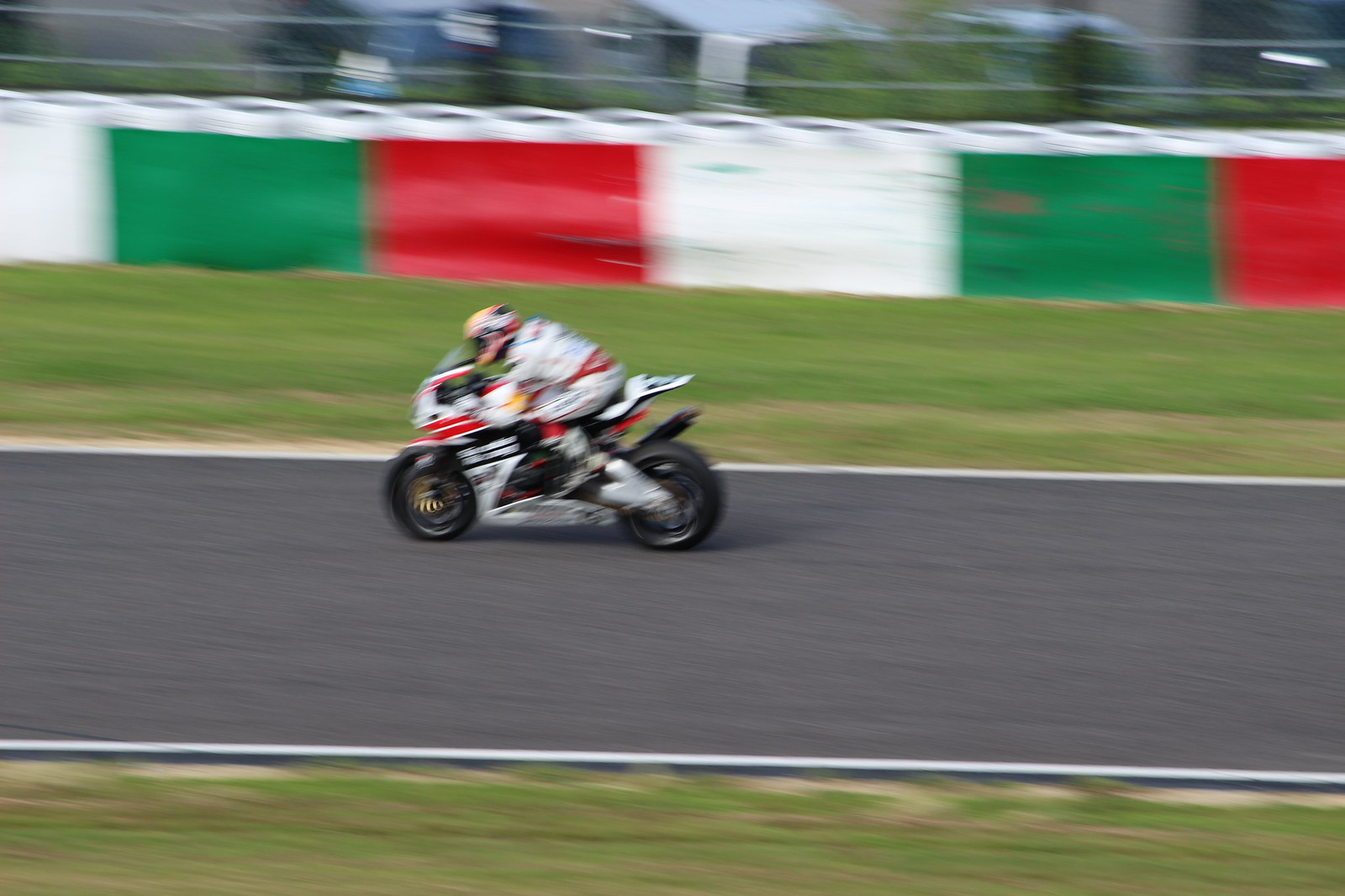This photograph captures a professional motorcycle rider in full gear, including a multi-colored helmet and predominantly white biker jacket and pants, racing at high speed on a gray racetrack. The white motorcycle, adorned with sponsor logos and red stripes, is captured mid-motion, creating a blur that emphasizes its velocity. The track, bordered by white lines, is flanked by patches of green grass on either side. In the background, a barricade displays a repeating pattern of the Italian colors—white, green, and red—adding a vibrant contrast. Beyond the barricade, partially visible structures lend depth to the scene. The wide landscape orientation of the photo accentuates the dynamic nature of the rider's motion as he races towards the left of the frame.